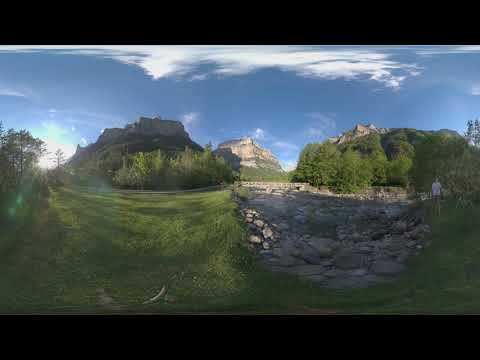The image captures a vivid natural setting, viewed through a fisheye lens, creating a slightly distorted, wide-angle perspective. Framed by a solid black border, the scene transitions from a grassy surface at the base to a sky dotted with clouds at the top. Central to the image is a meandering stream with a stone path, possibly a small brook or pond, which features a modest amount of water flowing through it. Alongside the stream, to the right of the center, stands a young man clad in a T-shirt and shorts, though he appears slightly out of focus.

On either side of the stream, there are hillsides adorned with trees, suggesting a dense forest surrounding the area. Distinctly, three prominent hilltops each host what looks like a fortress or castle, adding a medieval touch to the picturesque landscape. Near the setting sun, which glows from the left side of the image, one can observe the sky transitioning to shades indicative of late evening. Amid the tranquil scene, the untouched green space, strewn with stones and enveloped by nature's serenity, paints a serene picture of an idyllic outdoor environment.